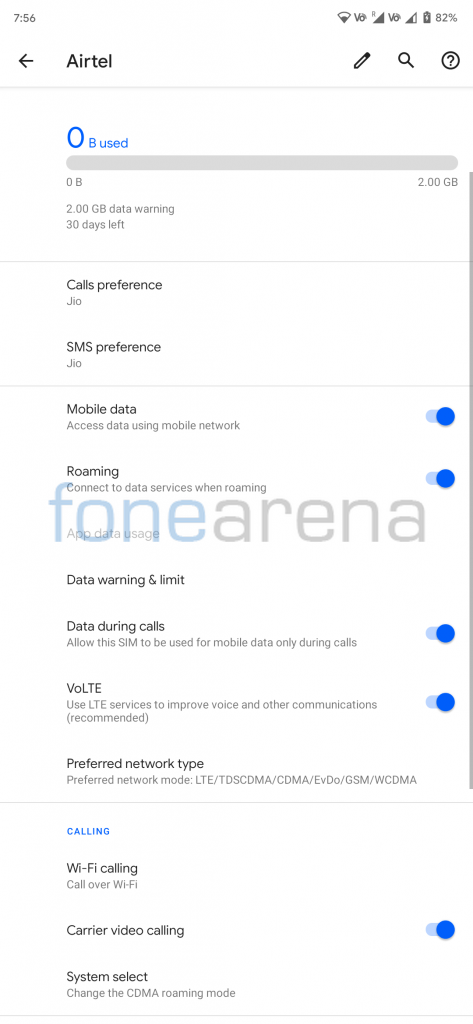An image of a mobile app's settings page titled "Airtel" is displayed on a white background. At the top, it shows "0B" indicating zero bytes have been used out of the 2GB data plan available, suggesting this could be a phone plan monitoring screen. A message warns that there are 30 days left in the current billing cycle. Multiple preference settings, such as "Calls Preference" and "SMS Preference," are listed, both labeled with "G-O" or "G-O-G-I-O." The "Mobile Data" option is toggled on, as well as "Roaming" and "Data During Calls." The "VOLTE" (Voice over LTE) feature, "Wi-Fi Calling," and "Carrier Video Calling" are all activated, indicating the user likely prioritizes seamless communication. Many toggles on the screen appear in blue, which could denote activated or enabled options. A back button is visible, along with the Airtel name and a watermark from "Fone Arena" spelled as "F-O-N-E." The detail within this image highlights the user's reliance on their mobile data plan and Wi-Fi connectivity.